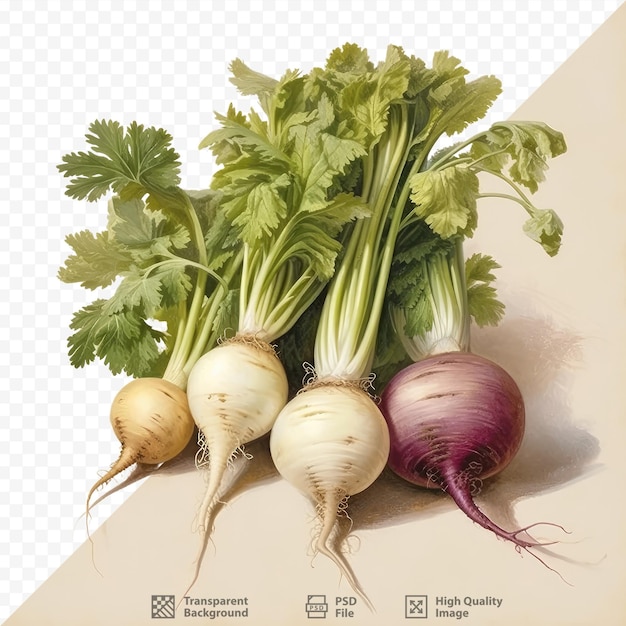In this illustration-style image, four radishes or turnips are depicted with intricate detail. One of the root vegetables is a tan color, two are off-white, and the last one exhibits a vibrant purple hue. Each of these vegetables is adorned with thick green leafy stalks, showcasing their freshness. They are arranged on an off-white surface, casting distinct shadows that add depth to the image. Above the stalks, the background features a white and gray checkered pattern, enhancing the overall aesthetic.

Beneath the vegetables, gray text and icons provide additional information. The first icon is a square box with arrows, accompanied by the text "High Quality Image." The next icon resembles a piece of paper with a rectangle, labeled "PSD File." The final icon displays a checkered pattern and stripes within a square, with the text "Transparent Background." The image boasts exceptionally crisp and clear quality, emphasizing the fine details of both the vegetables and the informative icons.